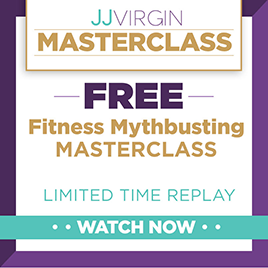**Descriptive Caption:**

A vibrant flyer advertises a "Free Fitness Myth-Busting Master Class" presented by JJ Virgin. The design features a visually appealing purple border with a combination of purple, teal, and gold colors. At the very top, a distinct gold-bordered square prominently displays "JJ Virgin Master Class." The word "Free" stands out in large, bold purple letters, immediately drawing attention. Beneath that, "Fitness Myth-Busting Master Class" is elegantly written in gold lettering. Below, in teal, it states "Limited Time Replay," with a "Watch Now" banner in white lettering set against the teal background. The overall design is professional and captivating, making the flyer both inviting and informative.